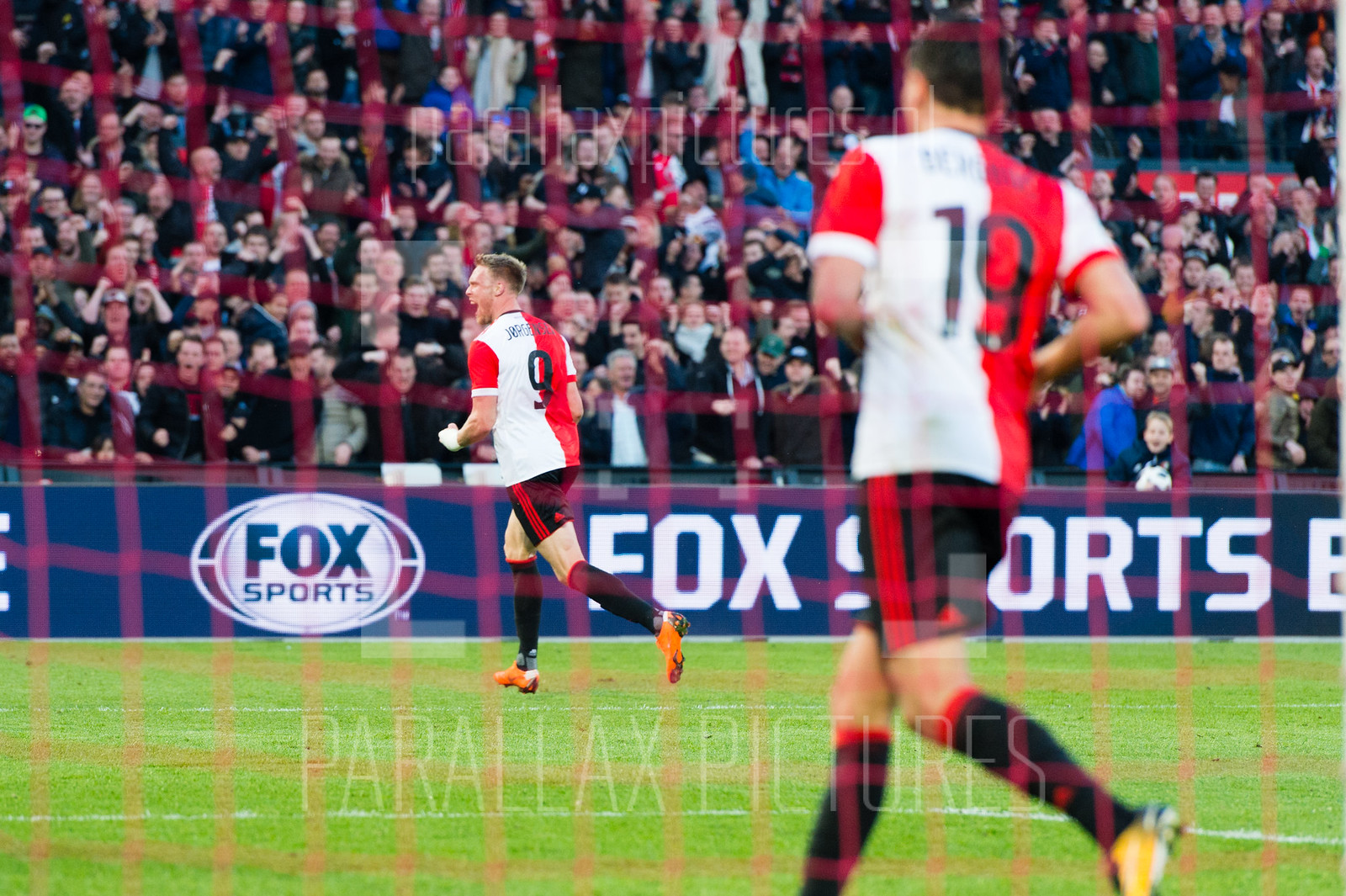The image captures a vibrant soccer match from the perspective directly behind the goal netting. Thin red netting lines streak across the entire scene. The background reveals a nearly full stadium of excited fans, many dressed in dark apparel, watching intently. A blue barrier, separating fans from the field, displays a prominent Fox Sports logo in an oblong shape followed by "Fox Sports" in large white text. On the lively green field, two male soccer players, wearing red and white vertically-striped jerseys, black shorts with red stripes, and black and red knee-high socks, are in motion. The player in the foreground is number 9, while number 19 is seen slightly further back. One player appears animated, possibly celebrating with a fist pump and an open mouth. Near the bottom of the image, "Parallax Pictures" is written in white letters.